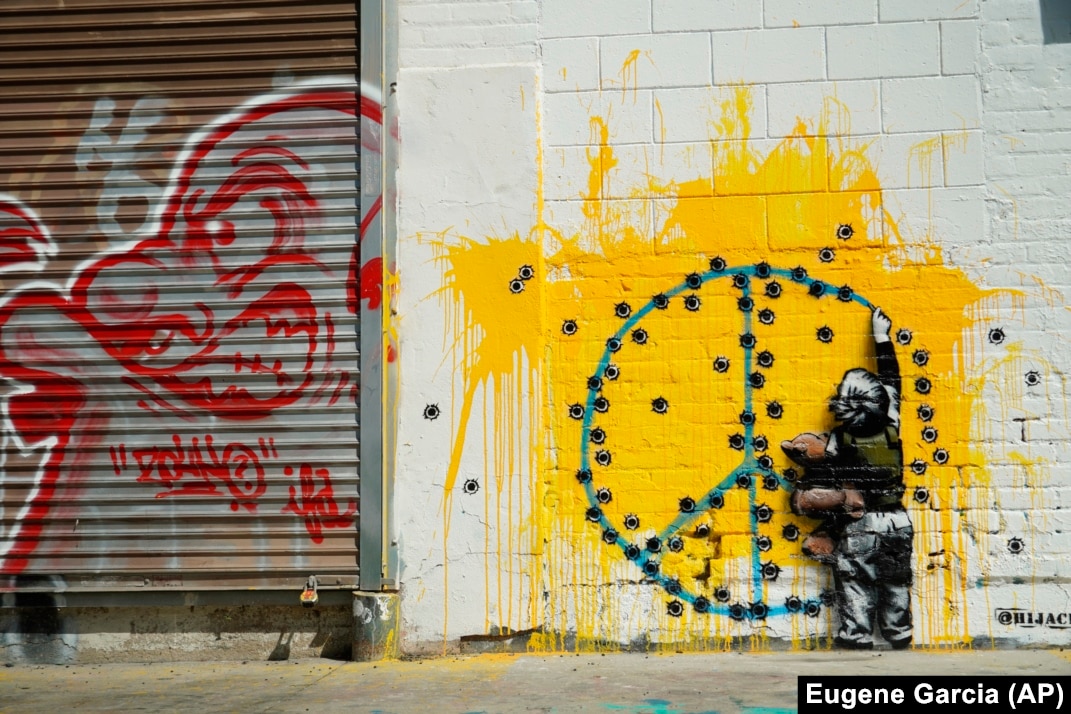The image depicts a wall with multiple finishes, divided into distinct sections. On the right, there is a white-painted section made of both large blocks and smaller bricks, which may indicate a previously bricked-in door. This section is notable for a dramatic splatter of yellow paint and a poignant piece of graffiti depicting a young boy facing the wall, holding a teddy bear in his left hand while drawing a peace sign with a blue marker in his right. The left part of the peace sign is unfinished, but intriguingly completed by a series of bullet holes scattered across the wall.

On the left side of the image, there is a metallic garage door, likely part of a business, featuring horizontal stripes and adorned with graffiti. The graffiti portrays a stylized, red-outline figure with an angry expression, including glaring eyes and a snarling mouth, clothed just down to the shirt level. The graffiti character appears to be a sketchy, rough outline, adding to the rebellious tone of the scene.

A sidewalk runs in front of the wall, marked by scattered paint sprays, further adding to the urban, gritty atmosphere of the location. The overall composition highlights contrast between the innocence of the child’s mural and the violence implied by the bullet holes, as well as the vibrant yet aggressive street art on the garage door. The artwork is signed "Eugene Garcia AP" in the lower right-hand corner, indicating the artist’s attribution.